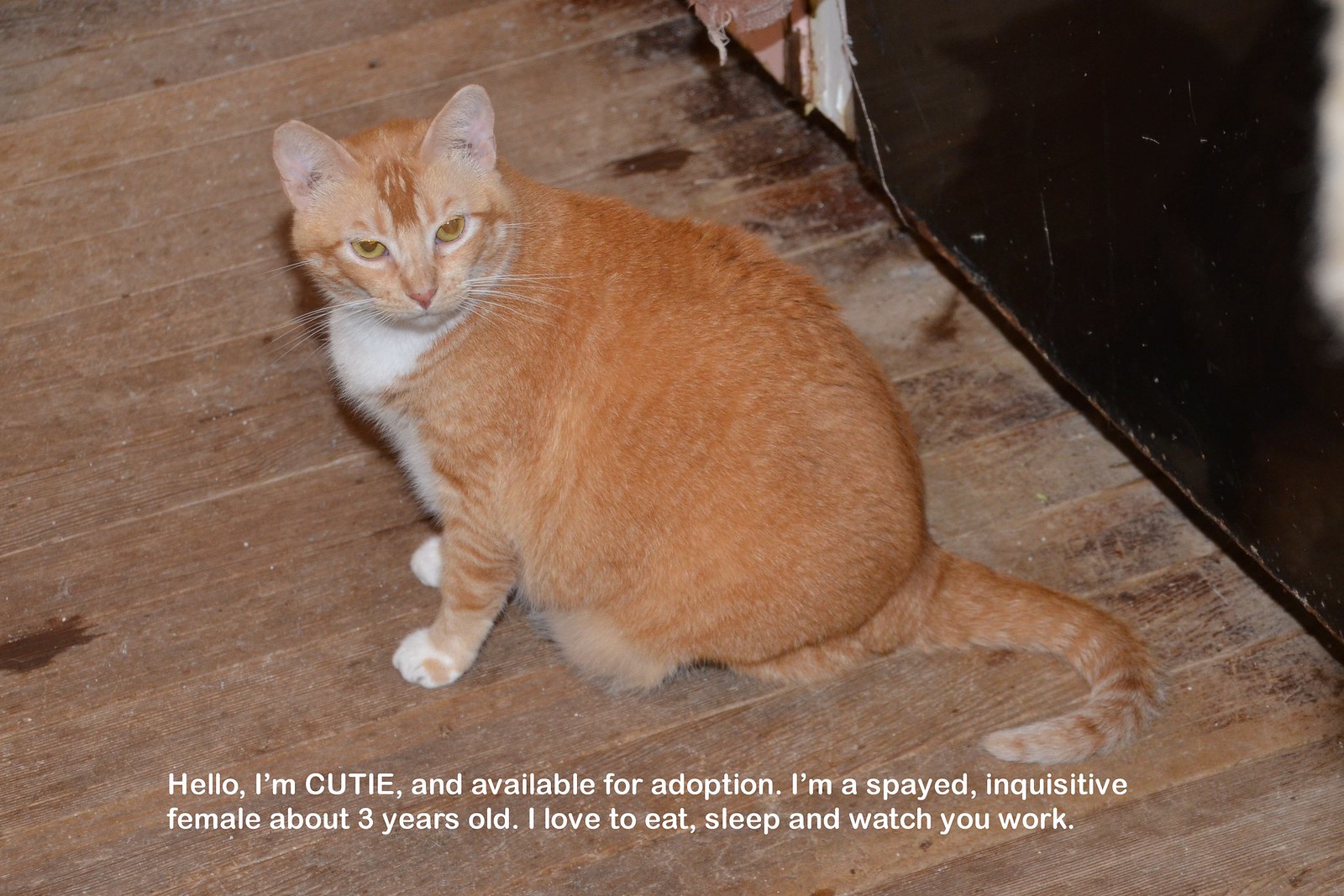A brown, short-haired cat with an orange-red coat and a white chest is sitting on a brown wooden floor in front of a black door. The cat, named Cutie, has raised ears and brown eyes, and is facing towards the camera with its body oriented to the left. Some brown items can be seen scattered on the wooden floor. The image includes white text at the bottom that reads, "Hello, I'm Cutie and available for adoption. I'm a spayed, inquisitive female about three years old. I love to eat, sleep, and watch you work." This appears to be an advertisement for Cutie's adoption, showcasing her endearing qualities and availability.